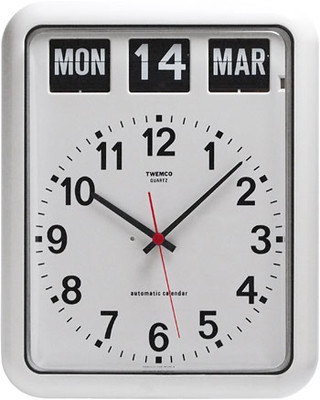The image depicts a square-shaped, white, plastic analog clock with rounded edges. At the top of the clock, there are three rectangular sections displaying the day, date, and month. The left section shows "Mon" for Monday, the middle section displays the numeral "14", and the right section indicates "Mar" for March, forming the date "Monday, 14 March". Below these sections, the brand name "Twemco" is visible, followed by the label "Automatic Calendar". The clock face features traditional black numerals from 1 to 12, with black hour and minute hands, and a red second hand, all connected at the center by a small red circle. The current time on the clock is approximately 10:08.